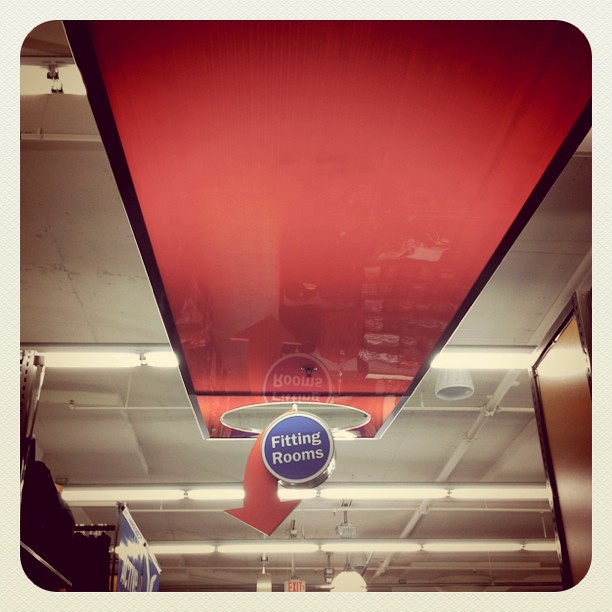The image depicts a high-angle view of a ceiling inside what appears to be a clothing store. The ceiling features white rafters and pipes, with four long, white fluorescent lights that are arranged horizontally across the scene, extending from the top to the bottom of the frame. Dominating the central area of the image, a red rectangular section is visible, reflecting light and adding a shiny contrast to the overall white and gray ceiling. Hanging from this red section, a blue, round sign with white text that reads "Fitting Rooms" is noticeable. This sign is bordered by a white outline and has a red arrow pointing downward. At the bottom of the image, a small, cream-colored "exit" sign with red text can be seen. On the right-hand side of the scene, there's a shiny, orangish door-like structure, while on the left, black metal racks are partially visible.